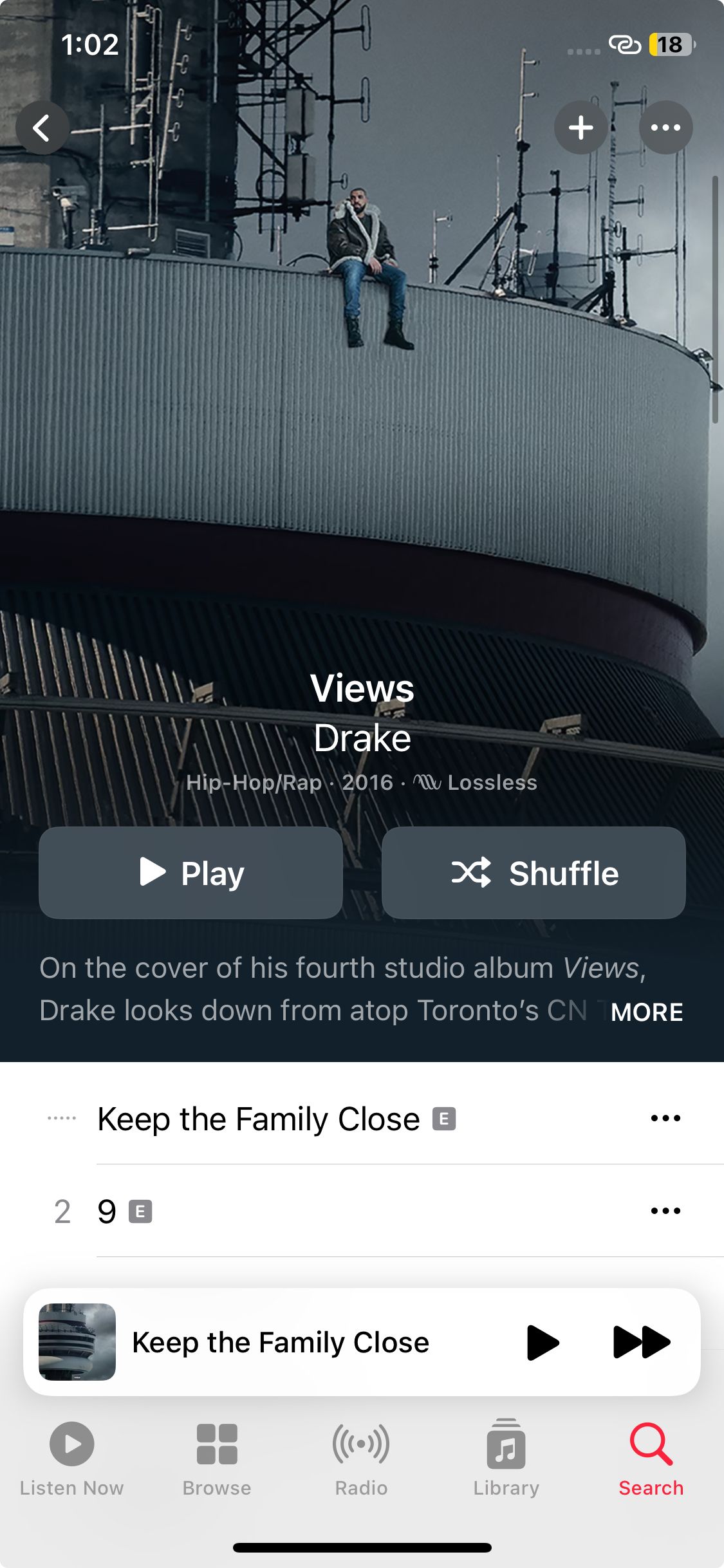This screenshot appears to be taken from a music streaming app, potentially Spotify, on a mobile device. At the very top, the time is displayed as 1:02, and the battery level of the device is at a critical 18%. To the left of the time, there is a plus sign, likely for adding the song to a playlist or creating a new one, and to its right are three dots indicating access to the settings menu.

The background image showcases the cover of Drake’s fourth studio album, "Views," featuring a massive building that resembles a stadium. At the very top of this building sits Drake, donned in blue jeans and a leather jacket with a fluffy collar, gazing contemplatively into the distance.

Beneath the image, the text reads: "Views Drake, Hip-Hop/Rap, 2016, Lossless." This is followed by options to "Play" or "Shuffle" the album. Further down, the partially visible synopsis states, "On the cover of his fourth studio album, Views, Drake looks down from atop Toronto's CN Tower..." with an option to read more.

The current track displayed, "Keep the Family Close," is highlighted, hinting it's possibly song number 2 or 9 on the album. Below this, there are navigation options labeled "Listen Now," "Browse," "Radio," "Library," with "Search" marked in red, indicating the currently selected option.